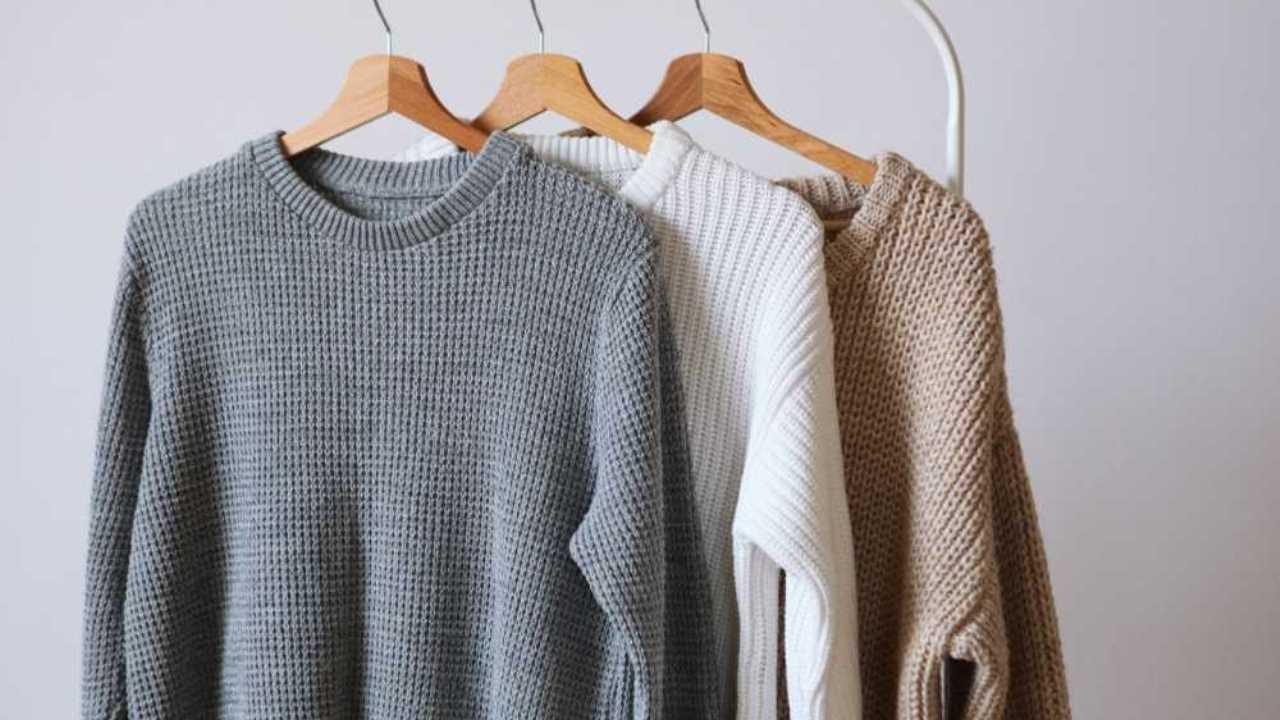This photograph captures a trio of medium-weight, ribbed men's sweaters hanging on smooth, wooden hangers. The hangers' metal hooks are just slightly visible below where they attach to the wooden section. Displayed against a lilac-gray, off-white wall, the sweaters are evenly spaced, suggesting a simple yet elegant store-like arrangement. The foremost sweater is gray and features a subtle mini check knit design, while the partially visible middle sweater is white and ribbed. The rearmost sweater is also ribbed and is a beige or light brown color. Each sweater is designed with a crew neckline, adding to their uniform appearance and warm, heavy feel. There is no text in the image, and the overall aesthetic is minimalist, highlighting the texture and color of the sweaters against a blank background.